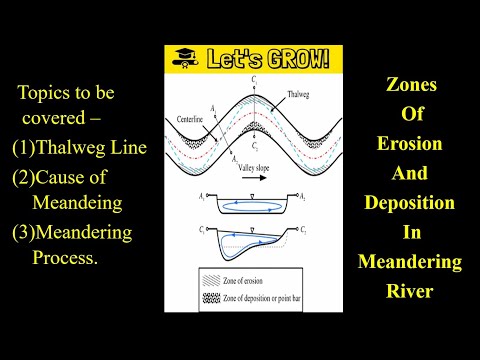The image is an illustration of the growth and dynamics within a meandering river, placed against a black background and framed by detailed annotations. At the top center of the white piece of paper features a vivid yellow banner stating "Let's Grow," accompanied by icons of a graduation cap and a rolled-up scroll, denoting educational content. This central diagram, reminiscent of a complicated elbow macaroni noodle with numerous joints, visually depicts the varied slopes, or valley slopes, and the associated zones of erosion and deposition—including a point bar—highlighting the intricate patterns within the river's meandering path.

To the left, written in yellow against the dark background, are outlined topics to be covered: 
1. Thalweg Line 
2. Cause of Meandering 
3. Meandering Process

On the right, text further describes the zones of erosion and deposition in a meandering river. The diagram also delves into cross-sectional views at various points labeled A and C, with a scale providing additional context. Each label meticulously identifies features such as depression areas where water accumulates and describes different river depths, contributing to a comprehensive understanding of the meandering river's behavior over time.